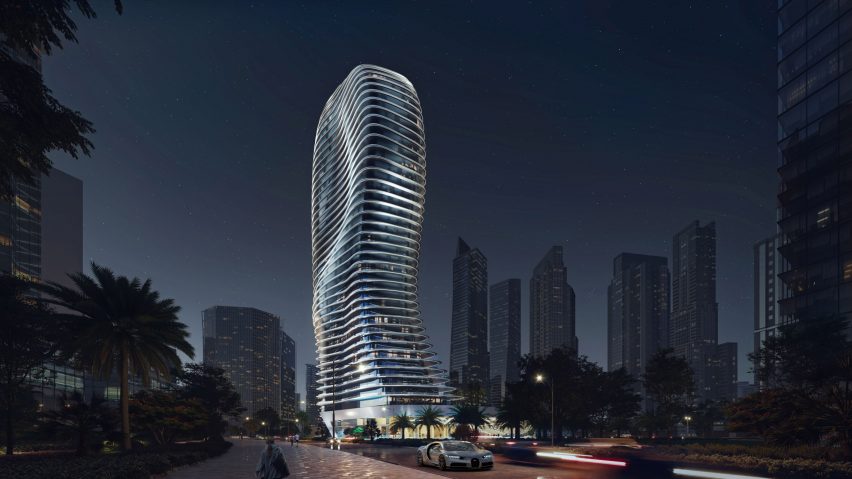This computer-generated urban nighttime scene showcases a highly innovative, curvy skyscraper prominently at the center. The futuristic structure, approximately 40 to 50 stories high, features protruding, ribbed floors creating a wavy, snake-like appearance. It is designed with a sleek whiteness that intensifies towards the base, illuminated to stand out against the darker, traditionally shaped high-rises in the background. The surrounding buildings are dimly lit, accentuating the central building's bright, sophisticated aesthetic.

The setting evokes a tropical vibe, possibly reminiscent of cities like Abu Dhabi, Miami, or Dubai, with palm trees scattered throughout. Cars, including a white sports car that could be a Ferrari, and streetlights populate the thoroughfare in the foreground. The night sky is a dark navy blue, with streetlights and building lights contributing to the ambiance. A few pedestrians, including a distinct figure in blue with a dark ponytail, can be seen walking along the glistening promenade, adding life to the vibrant, urban tableau.